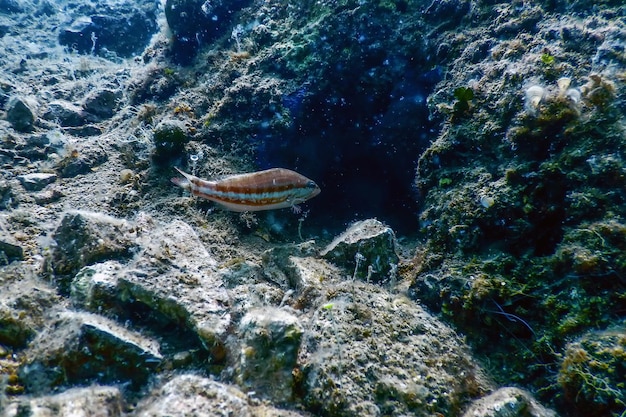In this detailed underwater scene, a photograph captures the serene and pristine aquatic environment. A small, light brown fish with a distinctive teal stripe running horizontally from its nose to its tail is the focal point of the image. The fish, positioned almost centrally, is swimming towards a small cave-like indent nestled inside a larger rocky formation. This cave, shrouded in darkness, adds an element of mystery to the photograph.

The underwater terrain is predominantly rocky, with the stones covered in a lush green algae that gives them a hairy appearance. Some moss and sandy patches are also visible, accentuating the natural and undisturbed ambiance of this underwater world. On the left side of the image, a red-orange-ish fish swims amidst the algae-laden rocks, adding a vibrant splash of color to the composition. Above, on the top left, a source of light penetrates the water, illuminating the rocks and enhancing the image's clarity, highlighting the textures and hues of the algae and rocks.

The water is remarkably clean and clear, devoid of any murkiness, silt, or suspended particles, allowing for an unobstructed view of the intricate details within the scene. The subtle play of light and shadows creates a captivating underwater tableau that portrays the tranquility and hidden wonders of marine life.